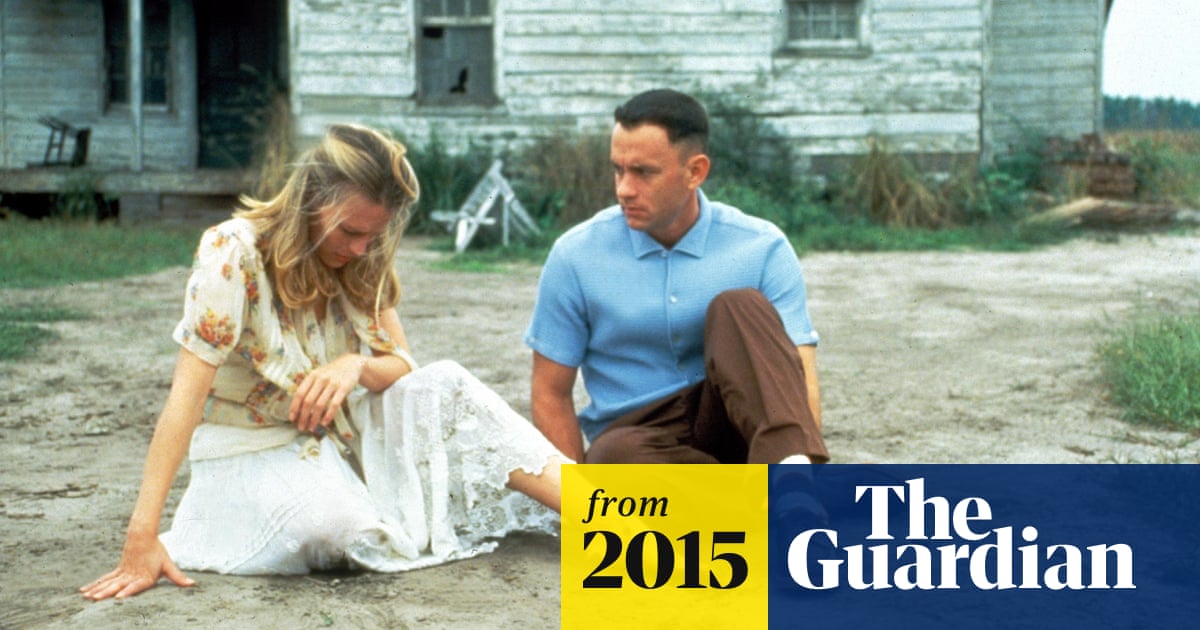This image appears to be a still from the movie *Forrest Gump*, featuring the characters Forrest Gump and Jenny. Both are seated on a dirt path in front of a dilapidated house with white faded wood siding and broken windows. The sky in the background suggests it's morning, and there's a knocked-over chair on the left.

In the foreground, Jenny is on the left, sitting with her right arm extended to the ground for support and her left arm resting gently on her upraised knee. She has sandy blonde hair pinned halfway back, a distressed expression, and is dressed in a white blouse with floral designs and a white, lacy midi skirt.

Next to her, Forrest Gump is sitting on the ground facing her, with a concerned look on his face. He has a short military-style haircut and wears a blue button-up shirt with brown pants. His arms rest beside him, and his knees appear slightly bent.

Overlaying the bottom right corner of the image is a caption. It consists of a yellow rectangle with the text "From 2015" in black, and next to it, a navy blue rectangle with "The Guardian" in white.